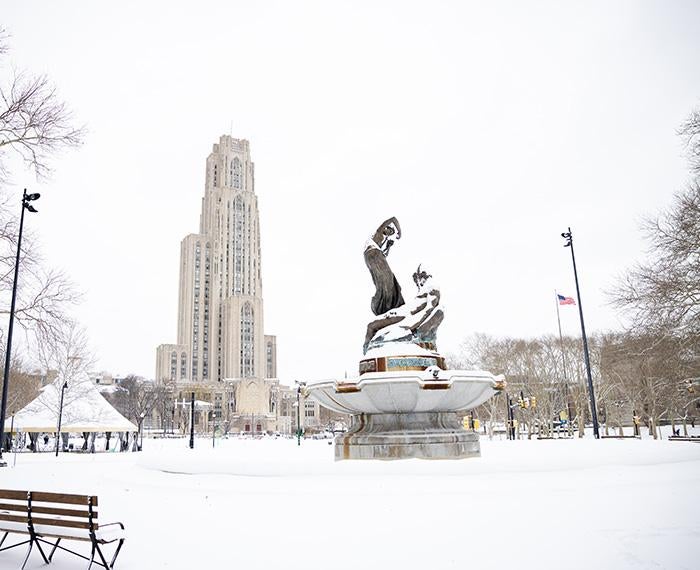This photograph captures a serene, snowy park scene dominated by an intriguing centerpiece—a statue. The statue, depicting a woman dancing atop a man, stands on a circular platform, possibly a fountain now dormant in the winter cold. The park is blanketed in pure, undisturbed snow, giving it a tranquil, desolate feel, further emphasized by the leafless trees that border the scene. In the bottom left corner of the image, a partially visible, empty bench hints at a place of contemplation. Rising in the background, a tall, beige-colored building with an art deco architectural style looms over the scene, reminiscent of the iconic tower at the University of Texas at Austin. To the back right, a flagpole with an American flag waves gently in the cold air. The image conveys a soft, monochromatic palette dominated by shades of white and gray, creating a stark contrast between the crisp snow, the grayscale statue, and the light-colored skyscraper.